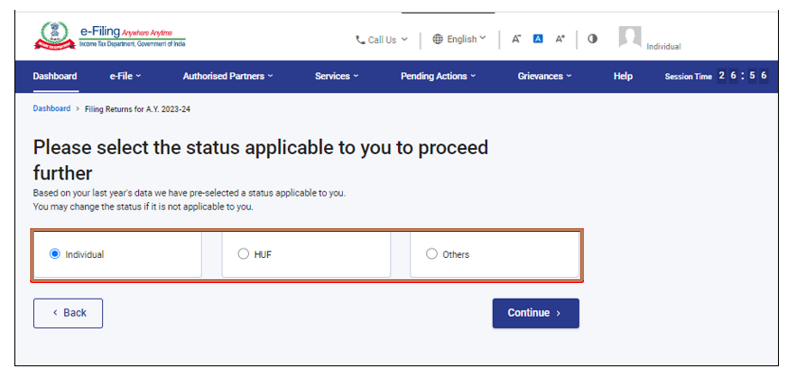This widescreen landscape image, appearing as a screenshot taken from a desktop or laptop computer, showcases the interface of the "e-Filing Anywhere, Anytime" portal by the Income Tax Department of the Government of India. The website features a sleek blue banner with several navigational buttons including "Dashboard," "e-File," "Authorized Partners," "Services," "Pending Actions," "Grievances," and "Help." The current session time displayed is 2656 seconds, indicating the user has been logged in for some time. The user, identified by the account name "Individual," is signed in with options for language selection and contact information available through dropdown menus.

The main content area prominently reads, "Dashboard: Filing Returns for AY 2023-24." Here, the site prompts the user to select their applicable status to proceed with the filing. It mentions that a status has been pre-selected based on last year’s data, though it may be changed if necessary. Below this message are three clickable buttons labeled "Individual," "HUF" (Hindu Undivided Family), and "Others," along with "Back" and "Continue" buttons to navigate through the filing process. The design features a clean white background with black text, ensuring readability and a user-friendly experience. This interface is clearly part of a common tax return service used in India, and the screenshot captures a user actively engaged in filing their tax returns for the assessment year 2023-2024.